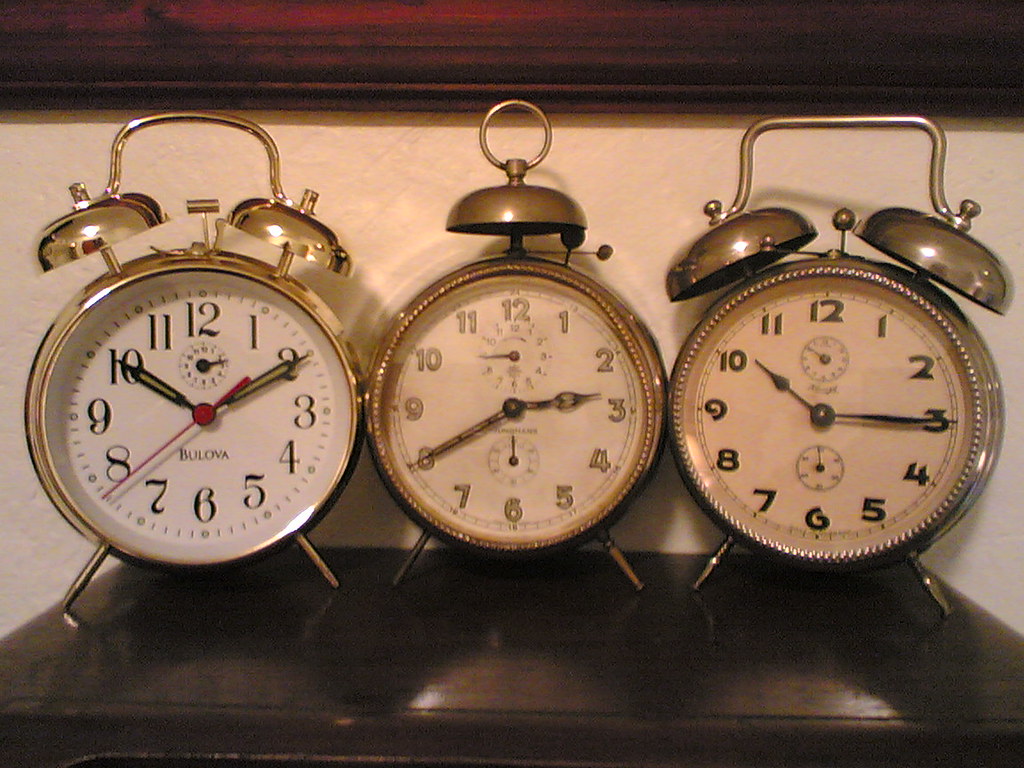The sepia-toned landscape photograph captures three vintage-style alarm clocks reminiscent of designs from the 1930s to the 1950s. Each brass-colored clock sits prominently on a shiny brown wooden table, spanning the width of the image. The clock on the left features bold gold numbers, a red second hand, and reads ten minutes after ten. The center clock, with a cream-colored face and softer beige numbers, displays the time as three-forty and has one large bell on top. The right-most clock shows fifteen minutes after ten and boasts two mini-clocks within its face, which are adorned with black numbers softer than those on the left clock. A wooden frame is visible just above the clocks, adding to the antique aesthetic. All the clocks appear to be ringing, though the image remains noise-free.